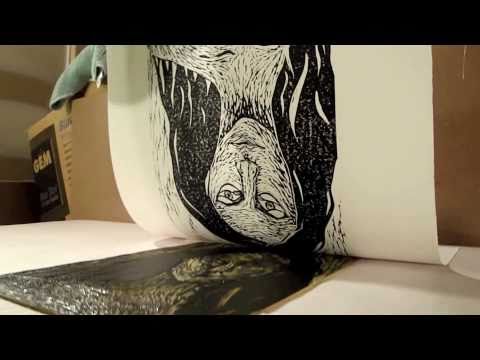This is a detailed photograph capturing the process of printing an inked etching. The main subject is an upside-down black and white image of a woman with long dark hair, large eyes, and a pronounced facial texture that could be wrinkles. The paper with the printed image is partially peeled off from a mold or plate beneath it, where a similar but darker image remains, suggesting fresh ink. The setting is a white tabletop with some background elements, including a cardboard box labeled "GEM" and a green towel. The process involves pressing the paper onto the inked mold to transfer the image, evident from the lifted paper showing the woman's face. The image appears to be cut off at the chest, and both images align closely, emphasizing the print's precision.